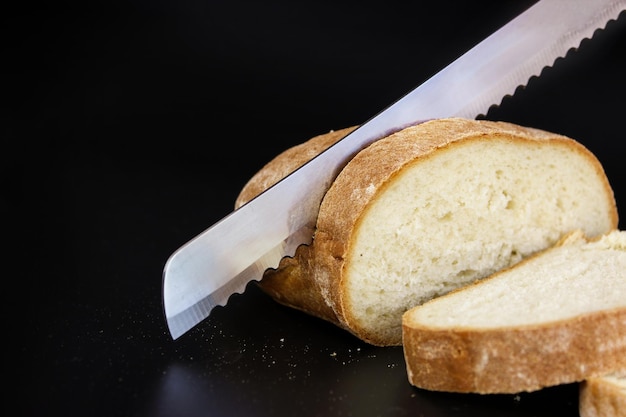In this landscape-oriented color photograph, a large serrated bread knife slices through a loaf of French bread. The background is solid black, providing a stark contrast to the golden brown crust and creamy interior of the bread. The loaf is positioned at an angle, with the knife entering from the top right corner and pointing toward the bottom left. The blade, which has a slight curve and a flat-ended nose, is partially embedded into the loaf, indicating the act of slicing. Two thick slices, already cut, lie close to the bottom right corner; one slice is fully visible while the other is partially cut off at the edge of the frame. Crumbs are scattered beneath the large piece of bread, adding to the realism of the scene. The photograph exemplifies food photography with a focus on representational realism, capturing the intricate details of the bread's texture and the moment of slicing.